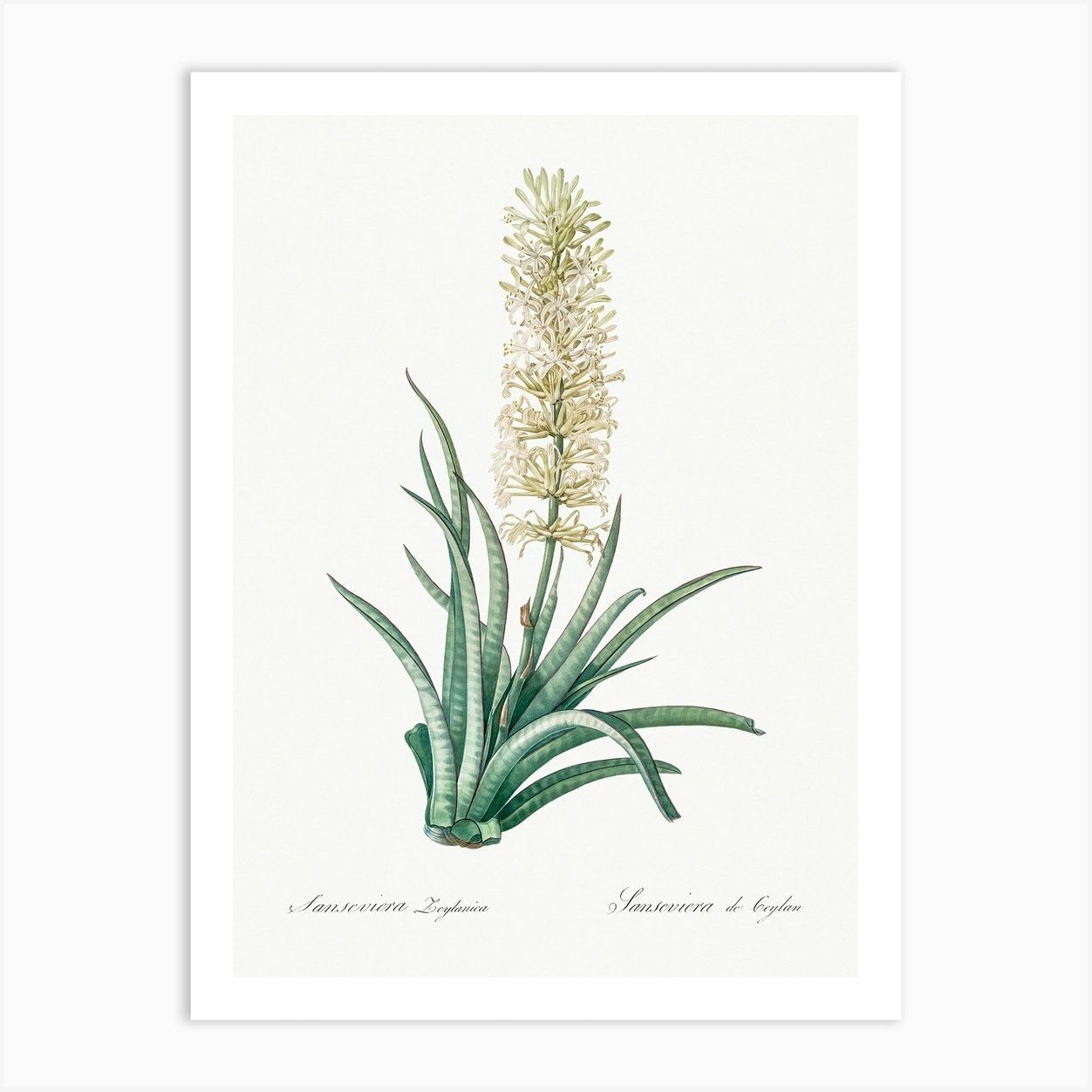The image is a detailed botanical illustration or painting of a tall plant set against a light blue background, framed by a white border. The plant features a long, woody stalk adorned with many small, white flowers that have long, thin petals and subtle touches of light green. Surrounding the base of the plant are numerous long, green leaves that resemble those of an aloe vera, characterized by distinctive white striped patterns akin to tiger stripes. At the bottom of the flowers, the names "Sansevieria lehanica" and "Sansevieria de Ceylon" are inscribed on the left and right, respectively, adding a scientific touch to this aesthetically detailed illustration.